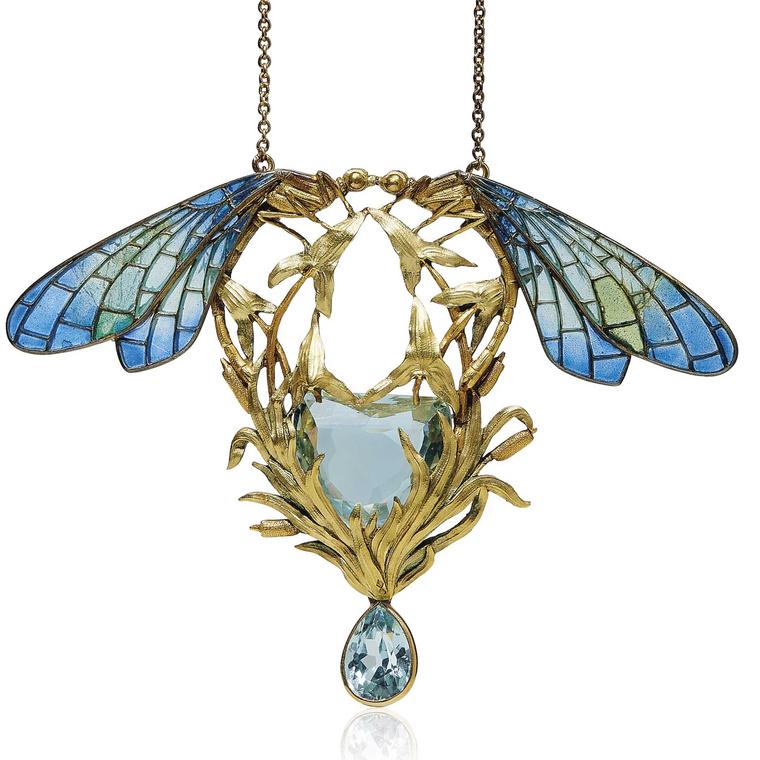This vibrant and professional image appears to be a product photo of an ornate necklace pendant, ideal for an online catalog or advertisement. The pendant is suspended by a gold or bronze-colored chain, branching into two segments at the top, each connected to a pair of intricately detailed wings resembling those of a dragonfly or butterfly. The wings feature a delicate gold webbing design, enhancing the allure of their light blue to bluish-green hues, reminiscent of stained glass. Below these wings, the pendant showcases an elaborate arrangement of golden, pointy leaves or petals, embracing a heart-shaped aquamarine gemstone at the center. Adding a final touch of elegance, a light blue teardrop-shaped gemstone, possibly enamel with intricate blue and white painted designs, dangles gracefully at the bottom.